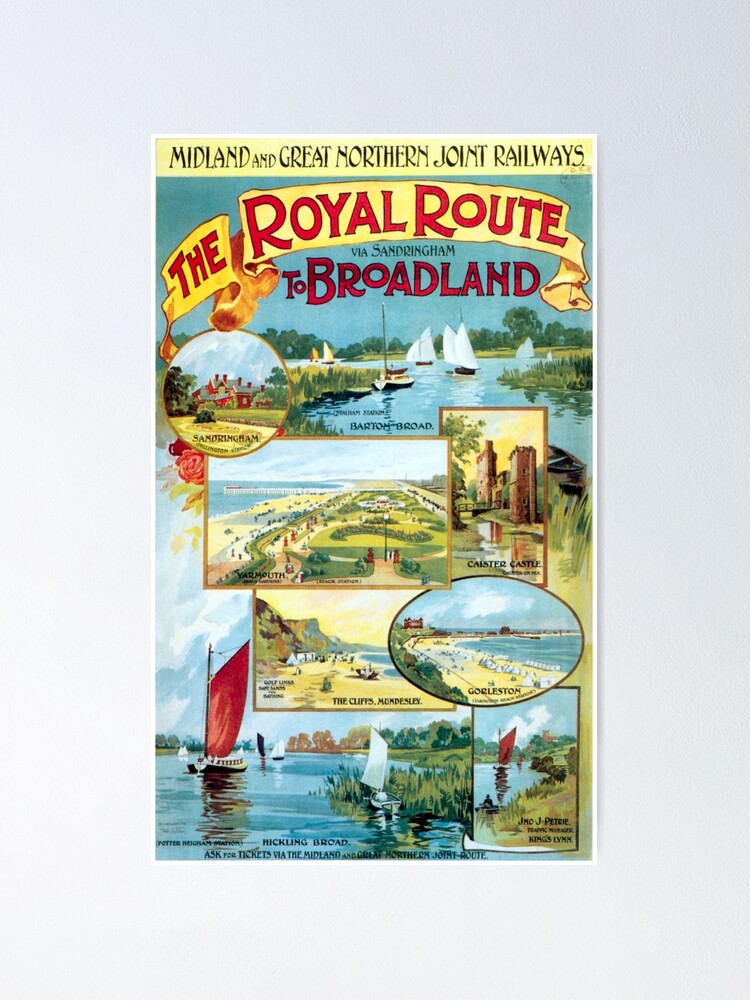The image is of an old flyer or poster with a predominantly white background, accented by a striking yellow band at the top. In bold black letters over the yellow band, it reads "Midland and Great Northern Joint Railways." Beneath this, a ribbon-like banner with a yellow background and red text proclaims "The Royal Route to Broadland via Sandringham." The main body of the flyer features colorful illustrations depicting scenes along the route: a vibrant blue lake with small boats, a circular inset of a farm with a red house surrounded by green grass, and an aerial shot showing land, sand, and sea. Another rectangular image showcases two tall, distant brown structures, while additional circle and square images highlight the coastline and waterways. Towards the bottom, there's a detailed drawing of a beach with people, water, and surrounding trees. Prominent throughout the flyer are multiple images of sailboats on water, including a striking ship with red sails. The color palette includes black, white, grey, red, yellow, blue, brown, and green, emphasizing the scenic and colorful journey depicted.